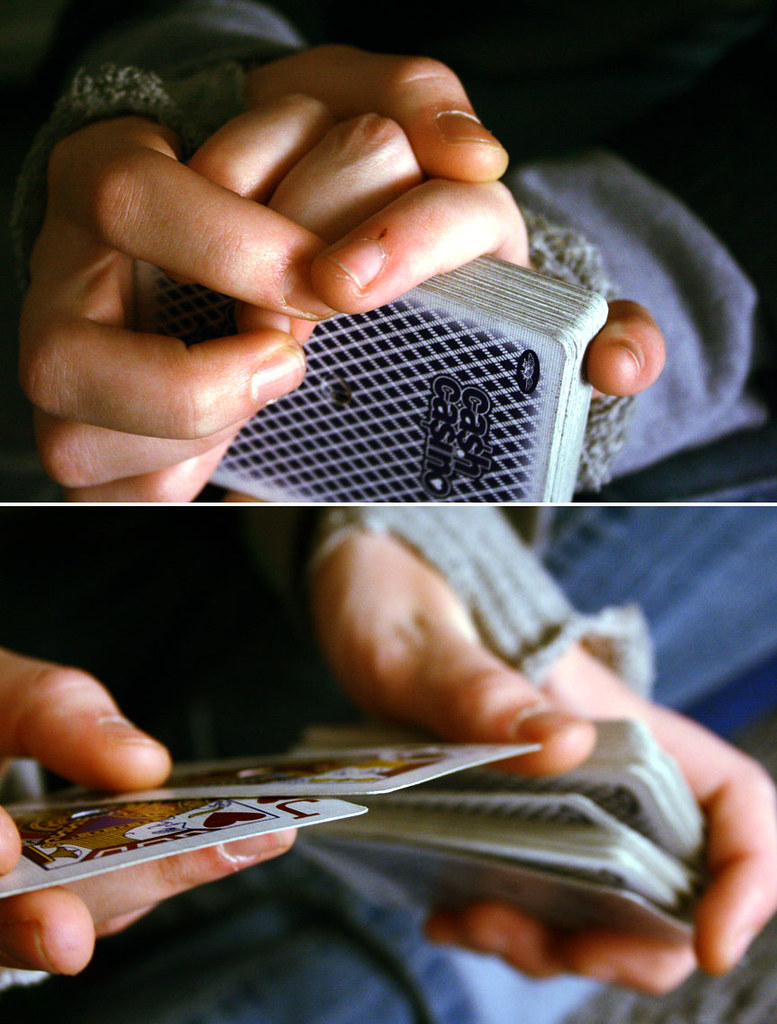The image consists of two distinct photographs arranged vertically. 

The top photograph features a pair of young adult or older child's hands holding a neatly organized deck of cards, as if ready to store them in a box. The fingers of both hands are visible, and a small cut with a bit of dried blood is noticeable near the nail of one finger. The person is dressed in a thick gray sweater, and a piece of gray fabric in the background likely represents their pant leg. The overall background is black, and the lighting is somewhat dim.

The bottom photograph shows the same person actively shuffling the deck of cards. They are still wearing the gray sweater, which has a thumb hole through which both the thumb and fingers protrude. In their left hand, they loosely grip most of the deck, while their right hand holds two cards that seem to have just been drawn from the deck. The individual's blue jeans, cuffed with a significant fold at the hem, are also visible.

The combined image captures a moment of casual card handling, providing a detailed view of the person's attire and actions within a slightly darkened ambiance.